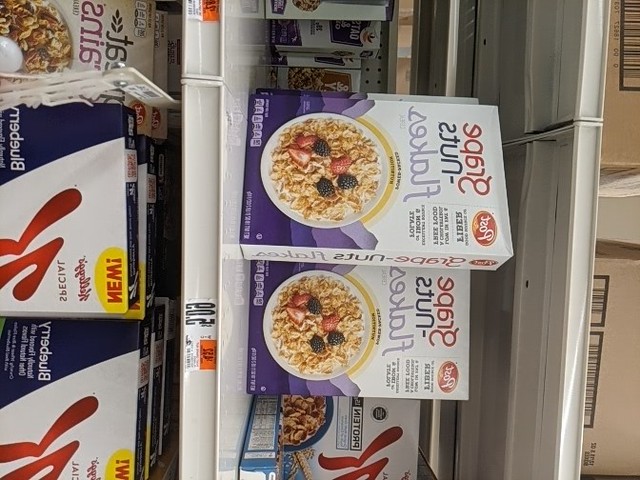This image, taken inside a grocery store, is oriented sideways to the right and appears to be mirrored, making the text reversed. Despite this, the setting is identifiable as a cereal aisle. The photo focuses on shelves stocked with various cereal boxes. On the top shelf, there are several boxes of Grape-Nuts cereal, priced at $5.09 each, which seems quite high for the size of the box. Below, on the bottom shelf, there are boxes of Special K Blueberry cereal. These elements dominate the frame, providing a concentrated view of the breakfast section in the store.